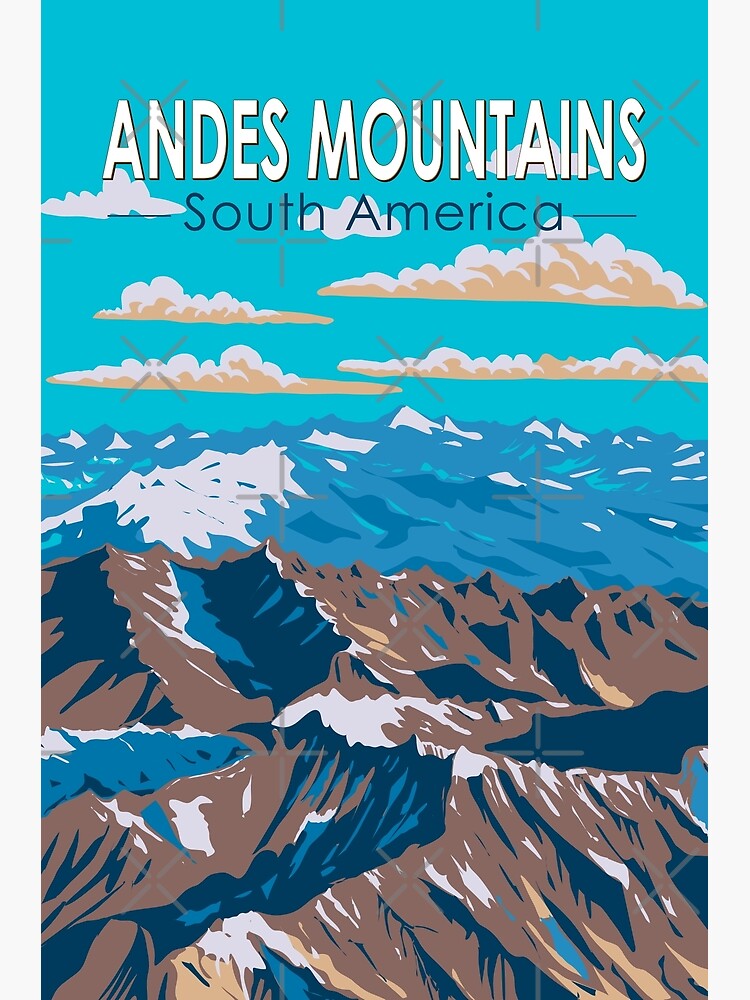This computer-generated poster depicts a vast, sweeping view of the Andes Mountains in South America. At the top of the rectangular image, "Andes Mountains" is prominently displayed in white, uppercase letters, followed by "South America" in thinner, navy-blue text beneath. The sky occupies the upper portion of the scene, boasting a light turquoise hue accented by seven clouds, some purely white and others tinged with a golden undertone. The Andes stretch across the lower two-thirds of the image, with the mountainous foreground bathed in warm light showcasing brown and navy shadows. Peaks in the background recede into a grayish wash, under soft, snow-covered summits. Light gray X's scatter throughout, suggesting a form of copyright marking.